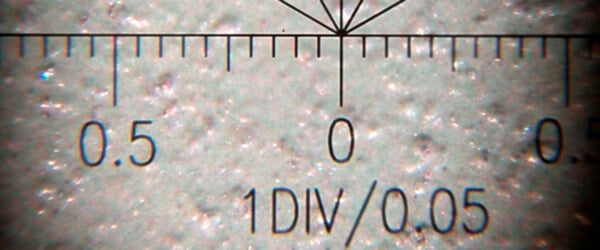This detailed image is an extreme close-up photograph of a metallic measuring stick, featuring a noticeably unusual, uneven texture with a silver-gray metallic hue interspersed with a pinkish bubbling texture, possibly indicative of rust or heavy use. The measuring stick, designed with hash marks and numbers for precision, is overlaid on this textured surface. Prominent black markings indicate measurements, with "0.5" on the far left, a central "0," and a partially visible number on the right side, starting with "0." At the bottom of the stick, printed in black, is the text "1 div / 0.05." The top of the image includes some diagonal lines cropping out, adding to the intricate detailing. This detailed, monochromatic image devoid of other colors or objects captures the wear and specificity of the measuring tool.